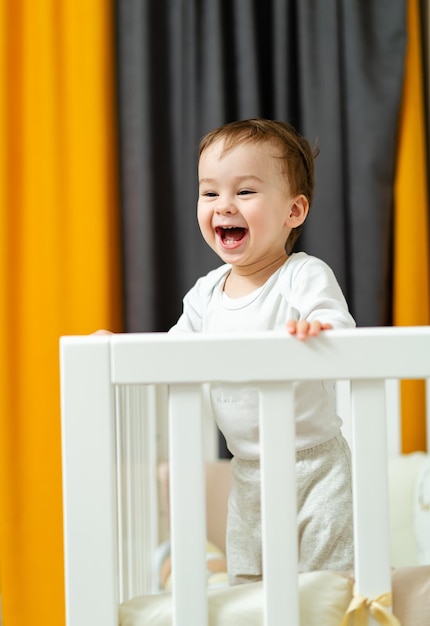This image depicts an infant standing inside a white crib, characterized by vertical and horizontal rails. The child, possibly around 10 months old, has dark hair, is Caucasian, and is wearing white pajamas, which include a white top and either white shorts or gray sweatpants. The baby exudes happiness, with an open mouth and visible top and bottom teeth as he laughs and smiles, seemingly at someone across the room. His hands grip the horizontal rails of the crib, and a gold ribbon is tied around one of the vertical rails. Behind the crib in the background are large drapes: a central dark gray or black curtain flanked on either side by goldenrod, yellowish-orange panels.